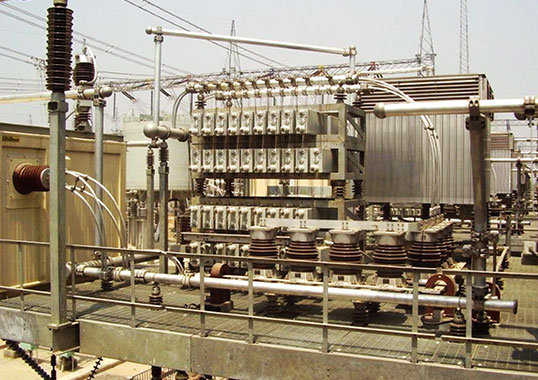This is a photograph taken outside at an electrical substation, capturing a complex array of metallic structures and equipment set on a raised metal platform. The focal point of the image is an intricate assembly of transformers and switches, surrounded by numerous pipes, metal compartments, buttons, and cylinders. Various electrical components, including resistors, diodes, and transistors, are visible, suggesting a high level of sophistication in managing electrical flows. A prominent yellowish-beige box, with wires extending from it, appears to connect to other parts of the system, possibly functioning as an electric converter. Suspended power lines stretch from the upper left of the image, receding into the distance toward the center top, while several metal-framed towers occupy the upper right-hand corner. The entire scene is set against an overcast sky, adding to the industrial atmosphere of this large-scale outdoor facility dedicated to electricity management.